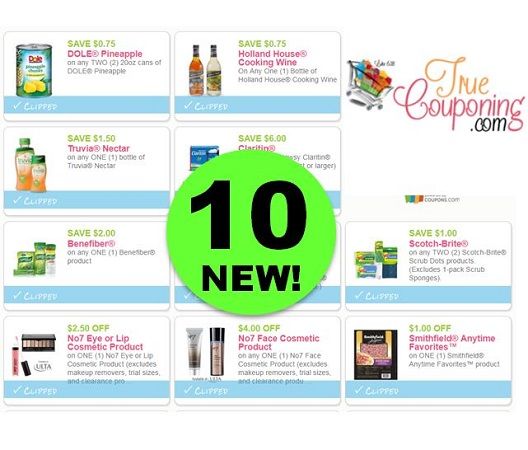This screenshot from TrueCouponing.com features a central lime green circle with the text "10 new" in black font. The image showcases 10 product photos arranged in 3 rows: two rows of 4 photos on the left and one row of 2 photos on the right. 

From top to bottom on the left side, the products displayed are: Dual Pineapple, Truvia Nectar, Benefiber, No7 Eye or Lip Cosmetic Product. The next items include Cooking Wine, Claritin, and the partially obscured product by the "10 new" circle, followed by the No7 Face Cosmetic Product. 

To the far left, the bottom two items are Scotch-Brite and Smithfield's Anytime Favorites. Positioned above the Scotch-Brite and slightly to the right is the TrueCouponing.com logo accompanied by an image of a shopping cart.